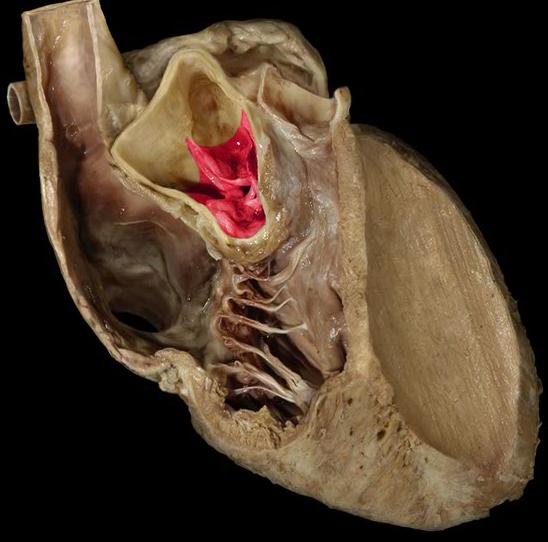This image, likely from a museum or a science book, depicts a sophisticated anatomical cross-section of an organ, possibly a heart or liver, either from a human or a large animal. The organ has a brownish exterior with intricate structures, including chambers connected by muscles and tissues, and visible blood vessels and lines. Part of the internal structure reveals a striking vibrant reddish-pink area. The organ is set against a completely black background, emphasizing its detailed features and isolating it within the frame. No date, text, or people are present, and the organ lies alone, detached, and potentially petrified.